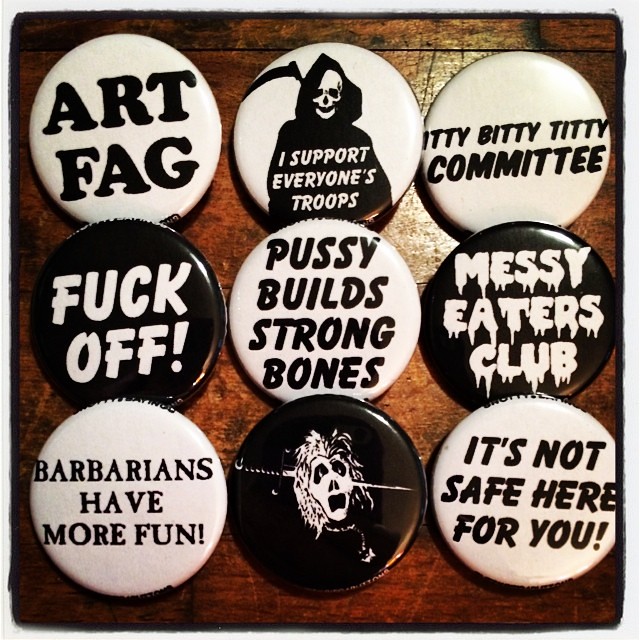In this image, there is a collection of nine black and white buttons neatly arranged in a 3x3 grid on a dark brown wooden table, suggesting either a personal collection or display for sale. Each button bears a unique slogan or design: 

1. Top left - A white button with "Artfag".
2. Top middle - A white button featuring the Grim Reaper, with the text "I support everyone's troops".
3. Top right - A white button with "Itty Bitty Titty Committee".
4. Middle left - A black button with "Fuck Off".
5. Middle - A white button stating "Pussy Builds Strong Bones".
6. Middle right - A black button with "Messy Eaters Club".
7. Bottom left - A white button saying "Barbarians Have More Fun".
8. Bottom middle - A black button depicting a figure screaming with a sword piercing through their head.
9. Bottom right - A white button with "It's Not Safe Here For You".

The buttons are laid out evenly, showcasing a mix of provocative, humorous, and subversive statements, indicative of a bold artistic style.